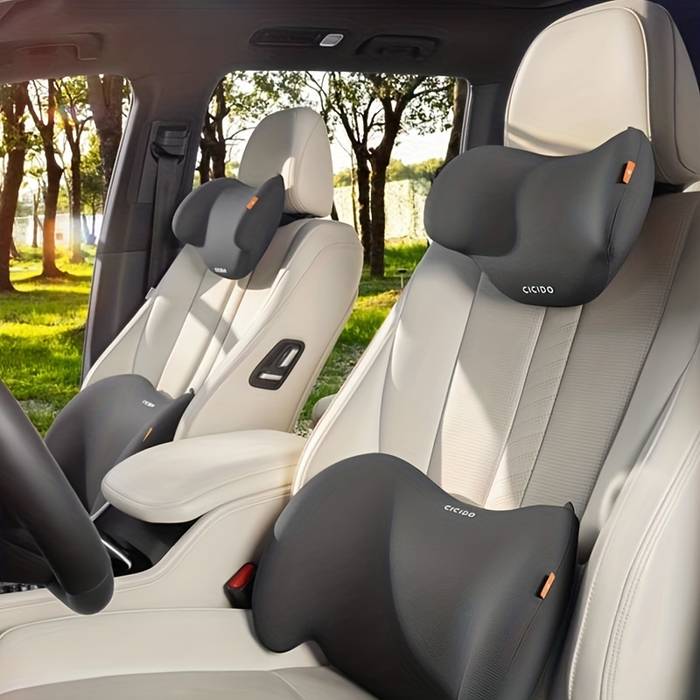The photograph captures the interior of a car, featuring the beige leather driver and passenger seats. Each seat is equipped with a CCDO (C-I-C-I-D-O) neck massage pillow attached to the headrest and a lumbar support cushion positioned at the lower back area where the seat belt is located. The word 'Secedo' is visible on both the neck pillows and lumbar supports, accompanied by a small orange tag on the right-hand side of each item. The interior of the car is a blend of beige and dark gray, with a partial view of the steering wheel and seatbelt. Outside the car, a serene landscape with a lake, trees, and green grass is visible, suggesting a peaceful, relaxing setting ideal for showcasing the comfort and relaxation these pillows promise during long rides.